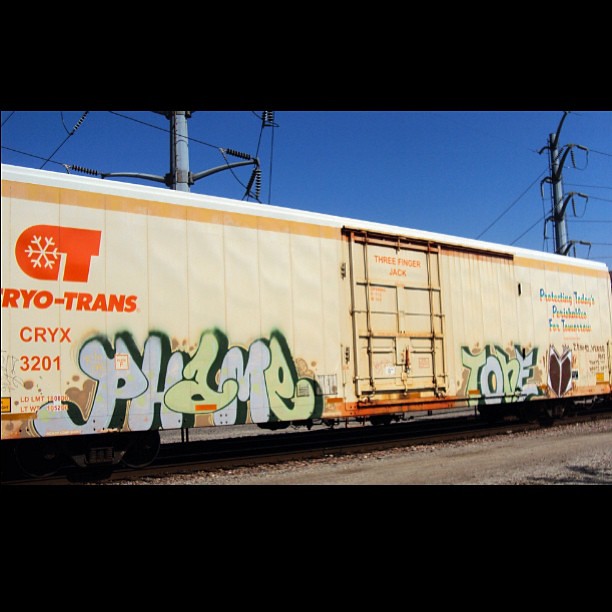The photograph captures a light tan train car, prominently displaying graffiti that reads "PHAME" in vibrant colors next to a heart shape, and "TONE" painted in blue and green near the center. The clear blue sky above has no clouds and is complemented by the presence of two tall electrical towers and wired telephone poles in the background. The train car features the partial brand name "RIO-TRANS" and the alphanumeric code "CRYX3201" below it, with "CT" and a symbol resembling a snowflake in a letter to the left. Though there is no date on the photograph, it is evidently taken during the daytime, and the camera angle slightly turned to the right reveals a view of the brown ground adjacent to the train. Black rectangles frame the image above and below, adding a sense of focus on the train car itself.